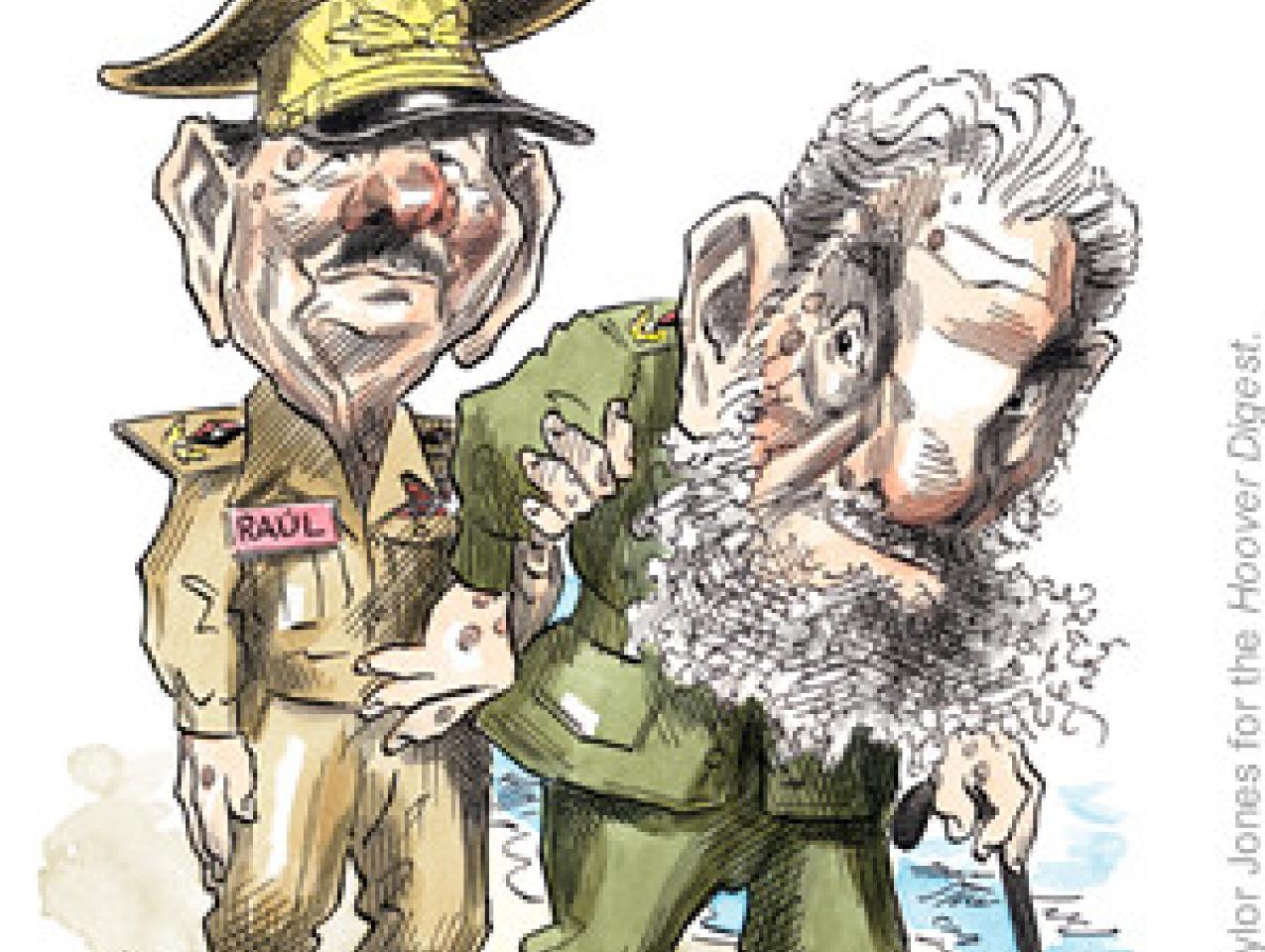The image is a vibrant political cartoon, likely created for the Hoover Digest, depicting an elderly Fidel Castro being escorted by his younger brother Raul Castro. Fidel, with his gray hair and beard, hunches slightly as he supports himself with a cane in his left hand. He wears a green military uniform, indicating his long years of service. Raul, whose name tag is visible on his khaki or light beige uniform, has black hair and a mustache. His hand firmly grasps Fidel's right arm, guiding him along in what appears to be a symbolic gesture of leading him out of his years of leadership. Both characters share exaggerated features, including large ears, big noses tinged with pink, and hands that seem overly large, covered with warts or moles. The setting seems peaceful, with pale watercolor tones and possibly a body of water in the background, emphasizing the calm yet poignant transition of power.